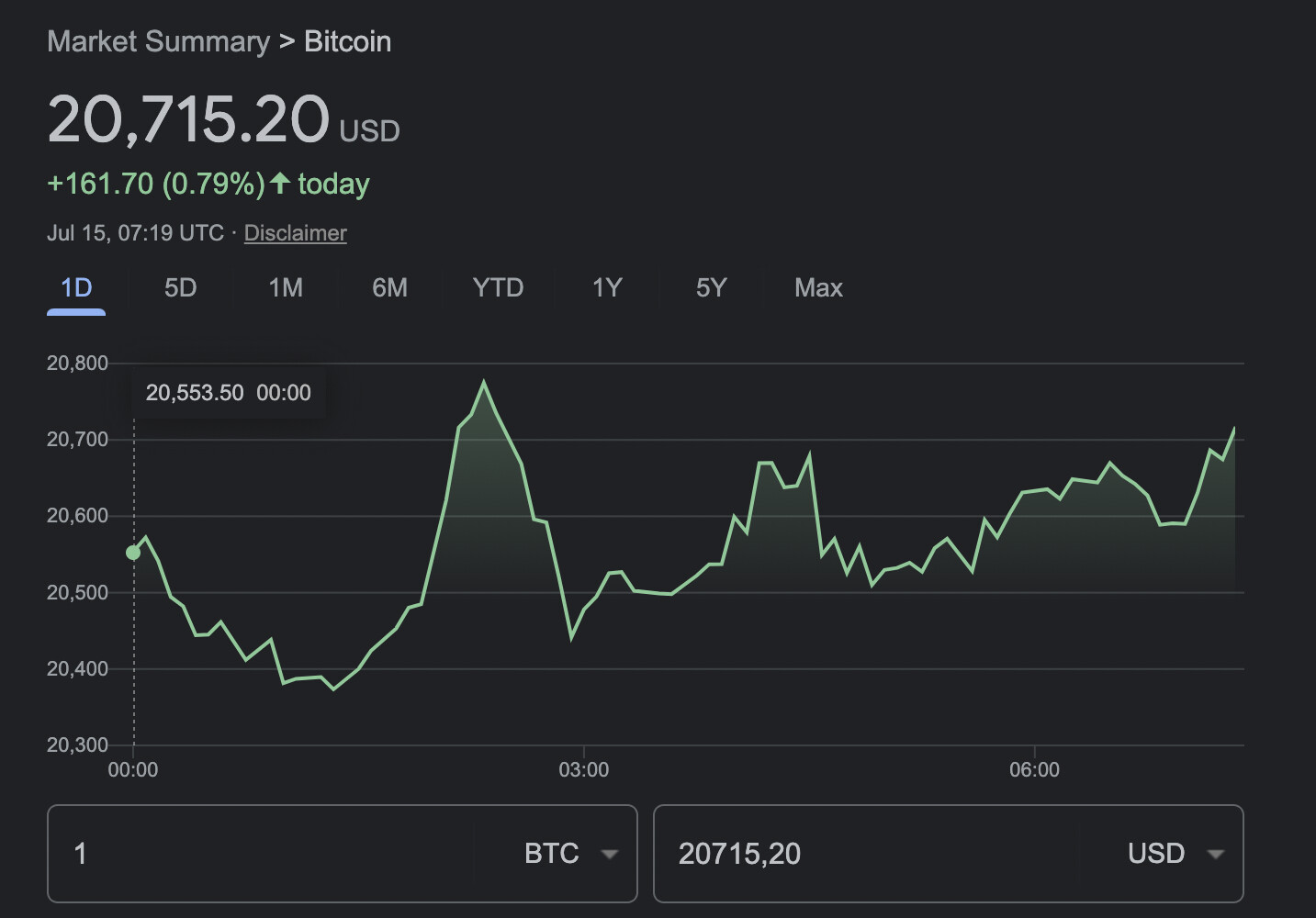This image features a detailed market summary for Bitcoin against a stark black background, creating a visually striking contrast. At the top, the header reads "Market Summary," with "Bitcoin" prominently displayed to the right. Below this title, the current trading price of Bitcoin is specified as $20,715.20 USD. The price has increased by $161.70 today, marking a 0.79% gain.

Capturing the date, the summary indicates the information is recorded on July 15th. Central to the image is a vivid green line graph depicting Bitcoin's price movement over the day. The selectable time intervals displayed above the graph include one day (1D), five days, one month, six months, year to date, one year, five years, and maximum timeframe, with the current view set to "1D" for a one-day overview.

The graph itself shows the price range for the day, with values fluctuating between a low of $20,300 and a high of $20,800. The price changes are traced over specific time points labeled in Coordinated Universal Time (UTC), giving a precise snapshot of intraday activity from midnight to around 7:19 AM.

At the bottom of the image, there is an input section where users can switch between displaying Bitcoin (BTC) in different currencies, currently set to USD. This comprehensive visual effectively encapsulates a single day's Bitcoin market activity, offering a nuanced view of its price dynamics.